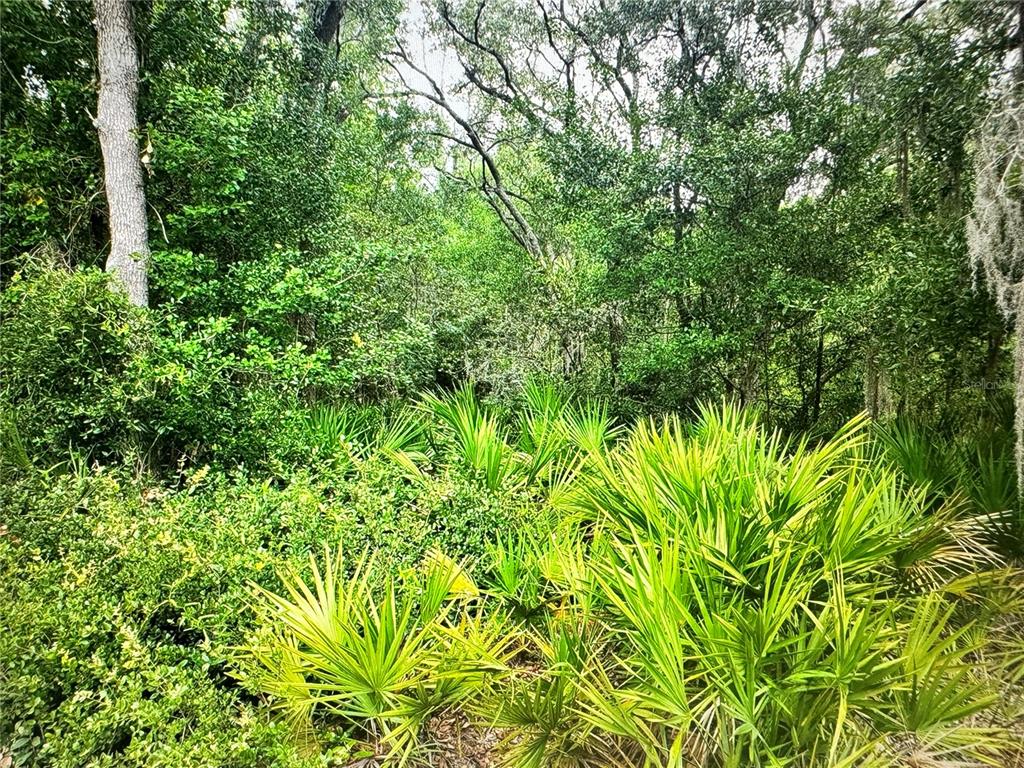This photograph captures an untouched slice of wilderness dominated by lush greenery. In the foreground, an array of bushes, shrubs, and varied foliage thrives, painting the scene predominantly in shades of green. Among the vegetation are low-growing, spiky-leafed plants, some with hints of yellowish-green hues. The middle ground features taller, dense bushes that blend seamlessly into the backdrop, which is populated with slender-trunked deciduous trees stretching upwards. The upper portion of the image reveals breaks in the tree canopy, exposing glimpses of a light gray sky. Notable elements include a gray and white tree stump in the top left and a subtle white flowery substance on the right. This verdant landscape, bathed in daylight, offers an impression of unspoiled nature with very little visible soil, emphasizing the area's rich and dense plant life.